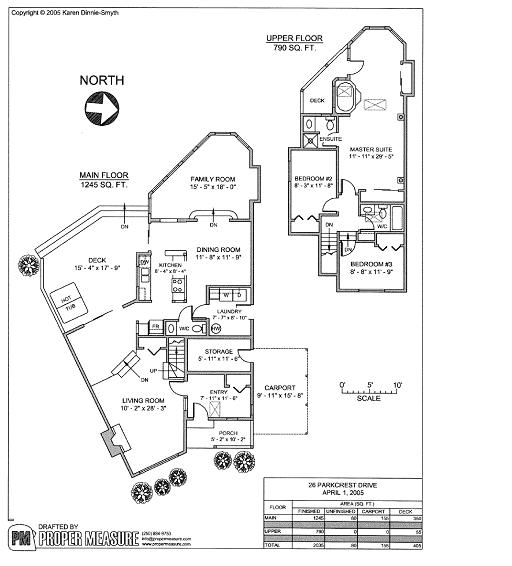A detailed blueprint of a two-story residential house, copyrighted in 2005, with a small, difficult-to-read name attributed to the drafter. The blueprint is labeled "Drafted by Proper Measure" and features a PM logo inside a measuring tape. 

The house design includes a carport on the bottom floor. The main floor, larger than the upper floor due to an expansive deck, encompasses various living spaces. The entryway, accessed through a small covered porch, leads directly into the living room. Adjoining the living room are the kitchen, dining room, and family room, all within a largely rectangular layout augmented by the deck on the side.

The upper floor is more compact, featuring three bedrooms and two bathrooms. Notably, the master bedroom includes a luxurious bathroom outfitted with a large bathtub or jacuzzi tub, offering a touch of opulence in this thoughtfully designed home.